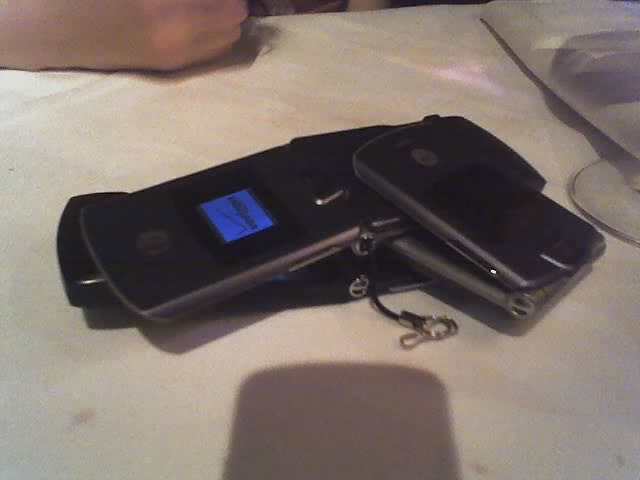The image features a stack of three Verizon-branded Motorola flip phones arranged on a white tablecloth. At the base of the stack lies an open flip phone. On top of it, another phone is positioned facedown and partially open, creating a clamshell-like appearance. The topmost flip phone is closed and rests on the middle one, with its blue LED screen turned on, displaying the Verizon logo. A small silver cable with a security clasp can be seen in the center of this arrangement. To the right of the phones is the clip mounting unit of a fold-over leather case, traditionally used to secure flip phones to a belt. Shadows cast by the devices, possibly from the person taking the photo, appear at the center bottom of the image. A clenched fist is visible at the top left corner, and a white object, possibly a plate or cutting board, appears at the top right corner of the frame, matching the color of the tablecloth. This intricate arrangement of old-school flip phones on an off-white background evokes a nostalgic sense of early mobile technology.